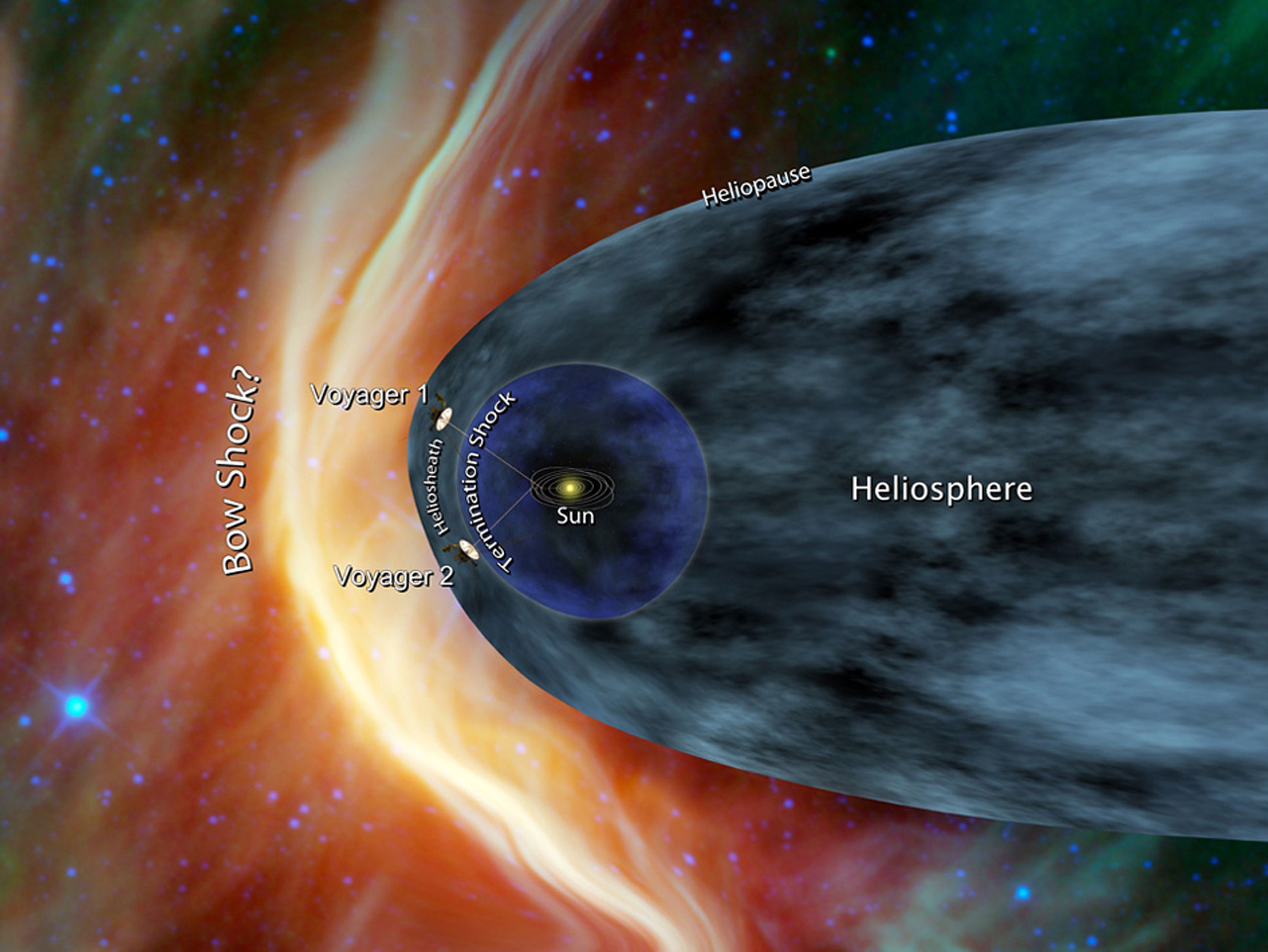This detailed schematic illustration depicts various cosmic phenomena and spacecraft within the heliosphere. At the center, the Sun is marked with a label. Surrounding the Sun is a blue circular region labeled "termination shock." Extending outwards from the Sun are lines indicating the positions of Voyager 1 and Voyager 2 spacecraft. The illustration also includes a larger enclosing oval labeled "heliosphere," with an outer boundary marked as "heliopause." On the left side of the image, there is an orange streak running vertically and an area referred to as "bow shock" with a question mark. The background features a starry sky with yellow and reddish-orange nebulae, enhancing the depiction of outer space.